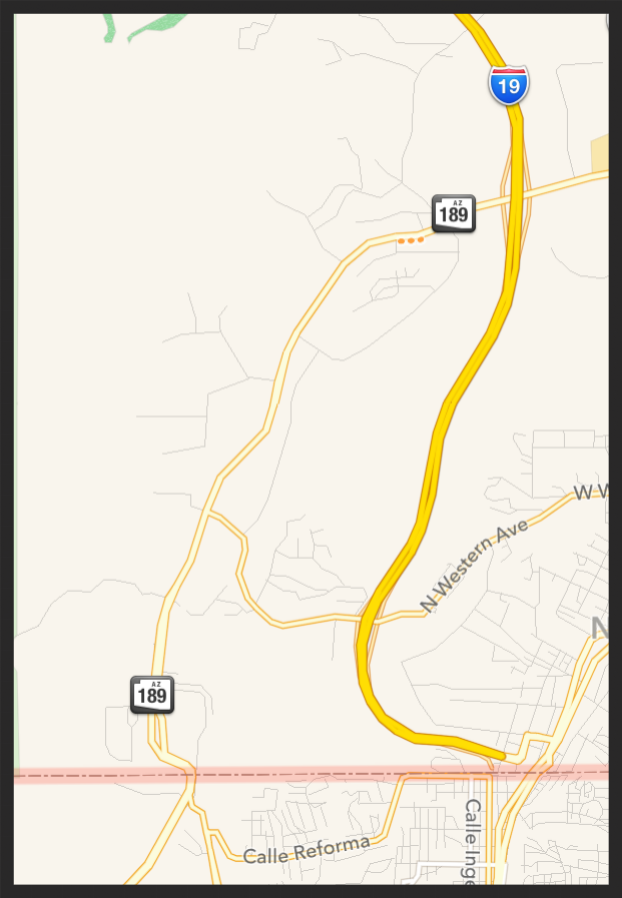This detailed map of a highway network prominently features Interstate 19 running north to south. Arizona Highway 189 is depicted traveling from the upper right corner, intersecting beneath Interstate 19, and continuing toward the state line at the bottom left corner. At the lower portion of the map, several smaller roads branch off from Highway 189, including Calle Reforma, a key avenue noted for residential and rural connectivity. Additionally, several unmarked smaller roads indicate further residential and rural development. The upper right corner shows Interstate 19 passing over Arizona 189, with visible exits and entry points facilitating traffic flow. Interstate 19's stretch concludes just before reaching the Arizona border, seamlessly transitioning into smaller local roads. A medium-sized highway, Northwestern Avenue, is shown on the lower right side of the map. The map is set against an off-white background, enhancing the clarity of the illustrated roadways.